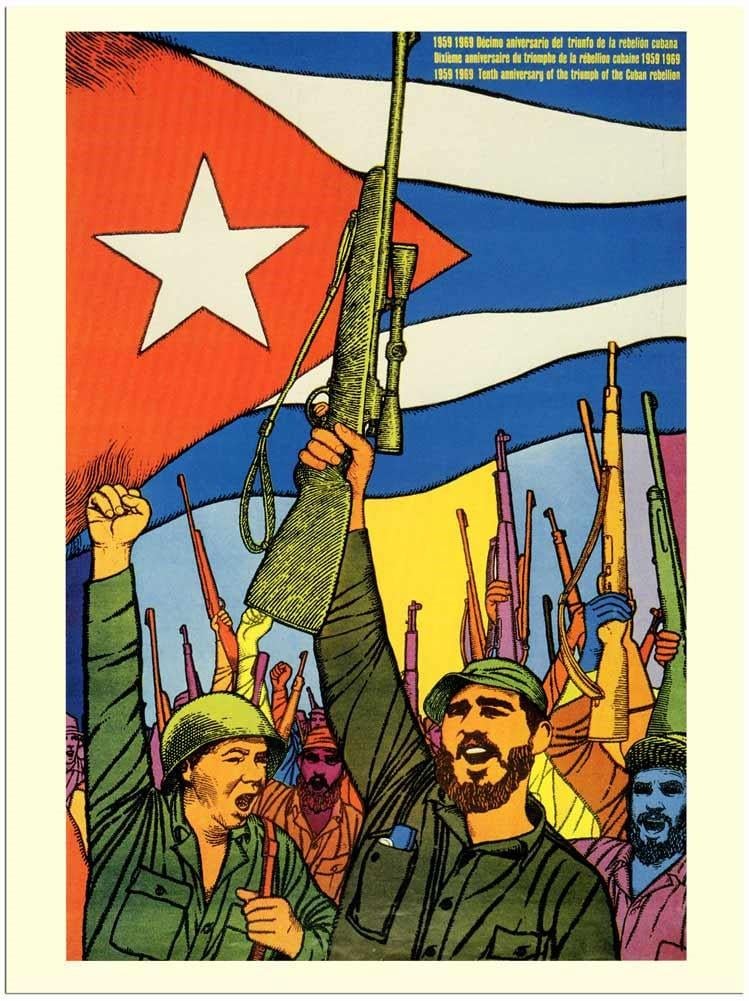This is an illustration styled as a historic political poster commemorating the Cuban Revolution. Dominating the upper portion is the Cuban flag, featuring blue and white stripes with a red triangle containing a white star, symbolizing the nation. Across the flag in the upper right corner, text reads "1959-1969, Decimo Aniversario del Triunfo de la Rebellion Cubana," translating to "10th Anniversary of the Triumph of the Cuban Rebellion."

Below the flag, a crowd of jubilant soldiers raise their rifles and fists in celebration. The centerpiece is a bearded man in a green button-up shirt and cap, clearly a figure of prominence and likely representing Fidel Castro. Surrounding him are other soldiers, one notable figure wearing a green shirt and a metal helmet, and others depicted in various colors including blue, orange, green, pink, and purple. The colorful depiction of the soldiers emphasizes the unity and diversity of those who fought in the rebellion. The overall style of the poster, with its vivid colors and cartoonish rendering, reinforces the celebratory and historic nature of the scene.